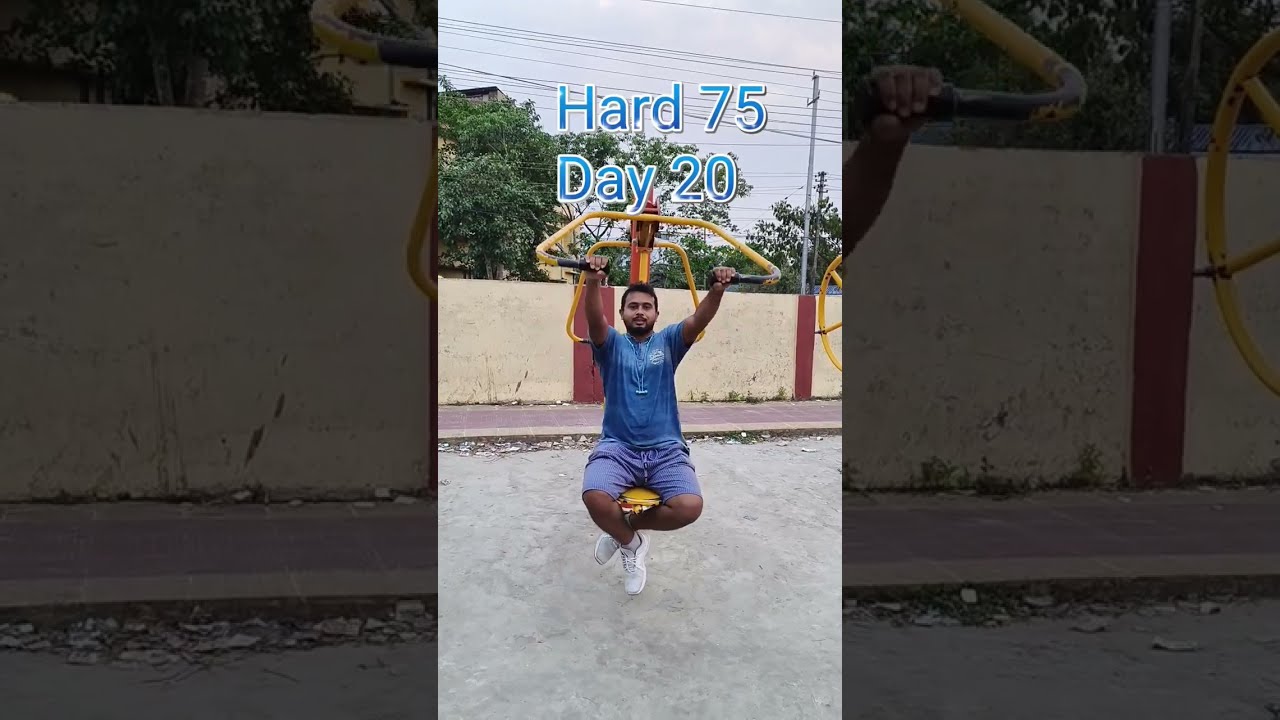The image features a man seated on yellow playground equipment, prominently centered in the frame. He is dressed in a dark blue t-shirt and blue jean shorts, with white sneakers. The man, who appears to be of Indian or Middle Eastern descent with dark brown skin, a beard, and black hair, holds onto yellow and black metal bars above him, possibly part of a weight machine or gym equipment. His legs are lifted off the ground, indicating an exercise pose. The equipment he is using seems to have an upside-down U shape, with some connection to a red component partially obscured in the image.

The surroundings are distinctly divided; the left and right portions are shadowy and grayed out, showcasing a cement wall, an old, beat-up road, and a walking area. The background reveals gray, cloudy skies, green trees, and telephone wires stretching across the scene. Behind the man, there is a tan cement barrier featuring a couple of vertical red stripes. Additionally, a red-brick colored sidewalk, somewhat washed out, lies beneath the barrier. 

Above the man, in a light blue teal font, the text "Hard 75, Day 20" is displayed, marking the upper center of the image. The overall setting gives an impression of an outdoor, makeshift workout spot.